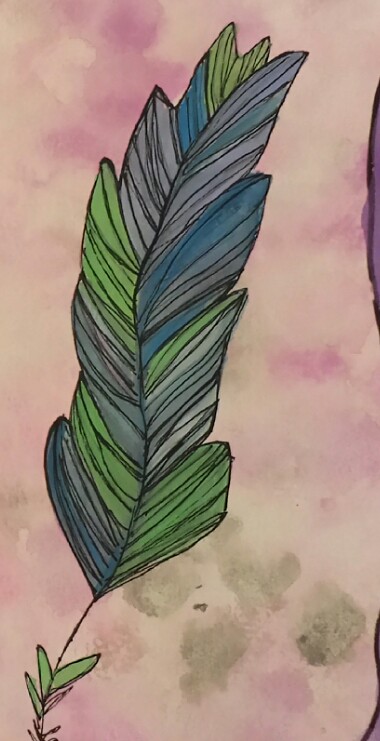This artwork is sketched on a piece of white paper adorned with muted shades of pink and green. The background, subtly blending dark and light pink hues, gives the piece a soft, pastel-like effect. On the left side of the image, the paper edges show slight wear with a faint hint of brown at the top and, more conspicuously, at the rounded bottom corner. In contrast, the right edge of the paper is straight and clean.

Prominently featured in the center is a meticulously drawn leaf. At the bottom, a slender stem connects to a small leaf adorned with three petite offshoots. Rising above is a large, feather-shaped leaf, intricately detailed with shades of dark green, teal, and gray. The leaf’s veins and outline are accentuated with fine black lines, enhancing its texture and depth against the softly colored background. This drawing elegantly captures the delicate beauty and structure of foliage through a blend of vibrant and muted tones.